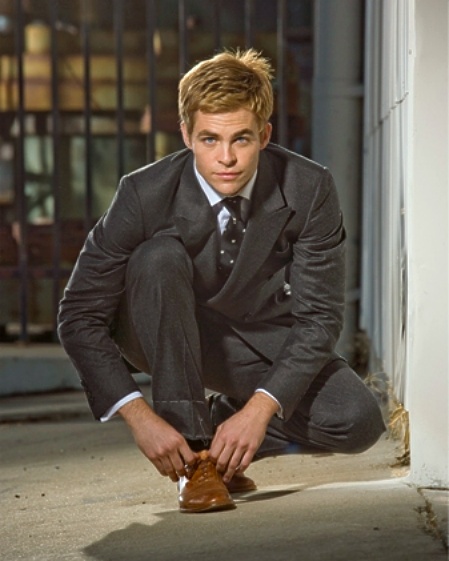This color photograph, possibly taken outdoors either at night or during the day, features a man dressed in a dark gray suit. He is bending down on the sidewalk, appearing to tie the shoe of an elderly woman, suggesting a moment of care and attention. The man, who has short brown or dirty blonde hair and a clean-shaven face, closely resembles a young Chris Pine, the actor known for portraying the new Captain Kirk. He is attired in a light blue shirt accompanied by a black tie adorned with polka dots. Behind him stands a metal or iron grate fence, adding a layer of texture to the background. This scene could easily be mistaken for a still from a movie, given its cinematic composition and the actor’s recognizable features.